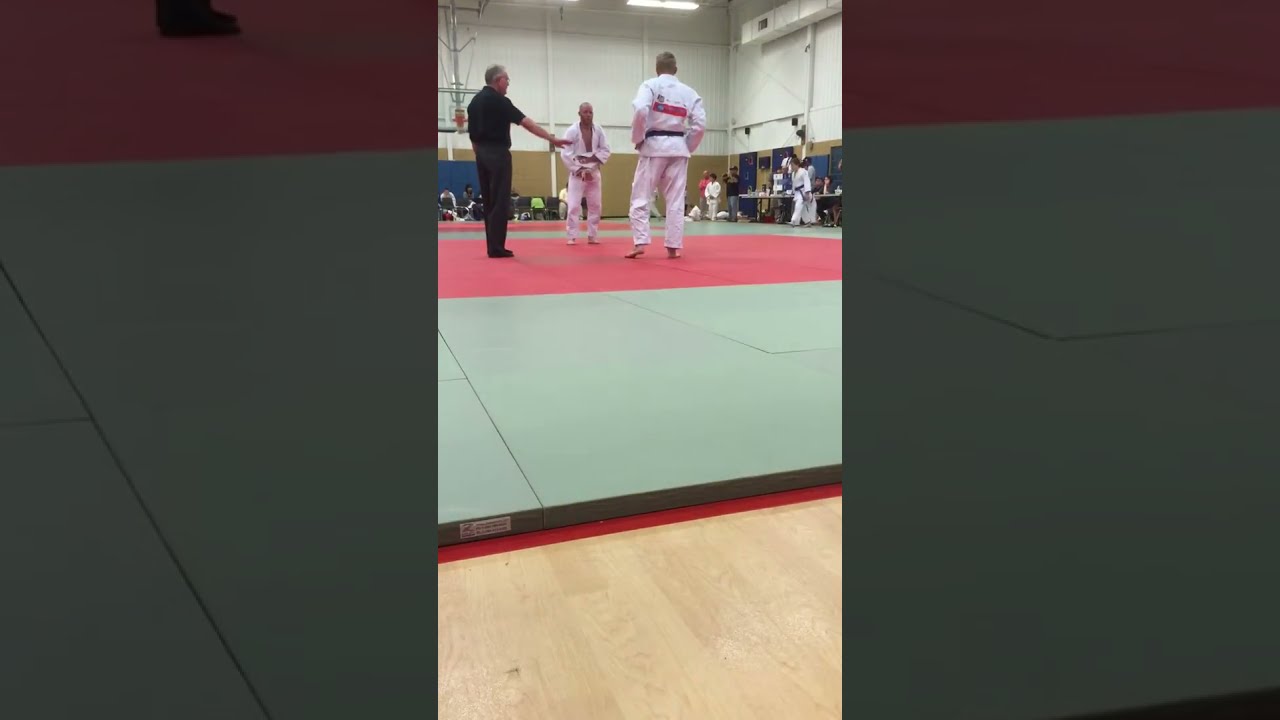The image depicts a vibrant scene of a karate match, likely taking place in a gymnasium or martial arts facility. The photo is taken from a low angle, capturing a large expanse of the lightly colored wooden floor at the bottom. Dominating the scene is a large mat composed of green with a red center where the two main fighters, both barefoot and in white karate uniforms, are engaged in combat. One fighter is distinguished by a blue belt. Their positions are somewhat centered toward the top of the image, where their figures are visible from the chest down, excluding their heads. 

In the upper corners of the image, there's a hint of the gym setting—noticeably a basketball backboard in the upper left—and a table on the far right with individuals who appear to be judges, also in karate uniforms. Various spectators and participants, all dressed in similar martial arts attire, encircle the fighting area, contributing to the dynamic, bustling atmosphere. The color palette includes shades of light brown, red, green, white, blue, lime green, and off-white, adding to the visual interest. There is no visible text within the image, and the overall arrangement feels slightly off-center, emphasizing the lively, somewhat informal nature of the event.